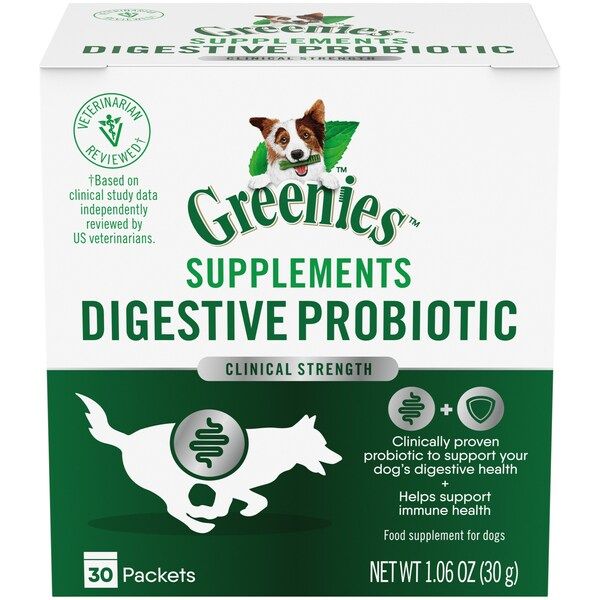This is a photograph of Greenies™ Supplements, presented in a white and green box designed for canine digestive health. The top half of the box is white, transitioning to green on the bottom. Prominent green text on the package displays "Greenies™ Supplements," specifying "Digestive," "Probiotic," and "Clinical Strength" in a metallic-looking section. The central image features a white and brown dog with brown spots around its eyes and ears, holding a green Greenies stick in its mouth, with a green mint leaf in the background. The "Greenies" logo, where the "i" is depicted as a bone with a small tooth, is positioned prominently above the dog. The packaging includes a symbol and the phrase "veterinarian reviewed," highlighting that the product is based on clinical study data independently reviewed by U.S. veterinarians. Additionally, a white outline of a dog and a digestive tract illustration adorn the front. The text at the bottom right reads, "Clinically Proven Probiotic to Support Your Dog's Digestive Health and Helps Support Immune Health," with the net weight of "1.06 ounces (30 grams)" and "30 packets" indicated on the bottom left.